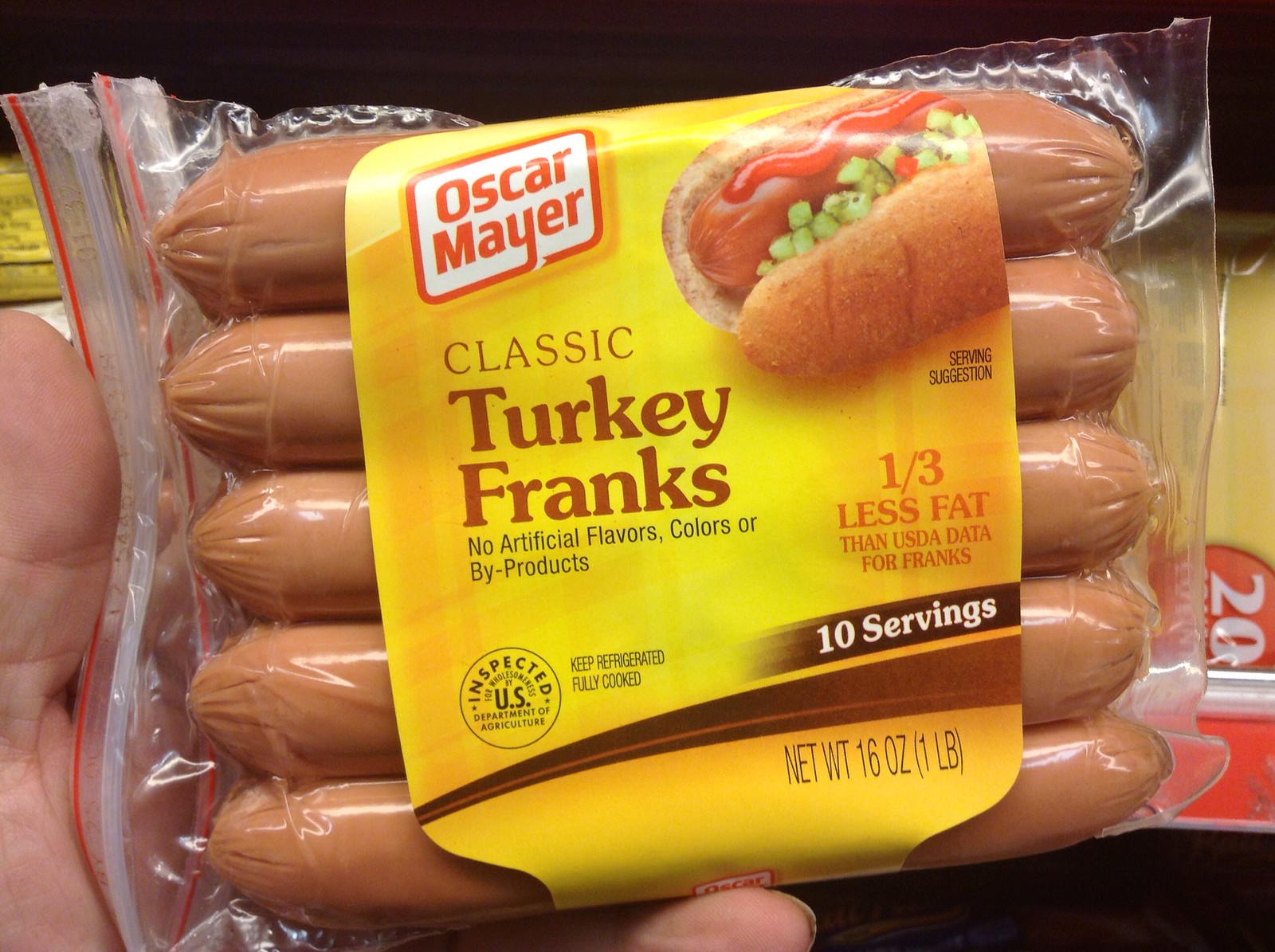The image features a package of Oscar Mayer Classic Turkey Franks being held by a person's left hand, with visible parts of their fingers and palm. The package prominently displays a yellow label in its center. In the upper left corner of the label, the Oscar Mayer logo is presented within a white box with a red border. To its right, a picture of a hot dog in a bun showcases a squiggly line of ketchup and chopped green vegetables, suggesting a serving suggestion. The label text, in varying shades of brown and orange, reads "Classic Turkey Franks," and highlights "No artificial colors, flavors, or byproducts," along with "One third less fat than USDA data for franks." Additional details include "Keep refrigerated, fully cooked," “Inspected U.S.,” “Net weight 16 ounces, one pound,” and “Ten servings.” Although five franks are visible through the shrink-wrapped transparent packaging, it is indicated to be a ten-pack.